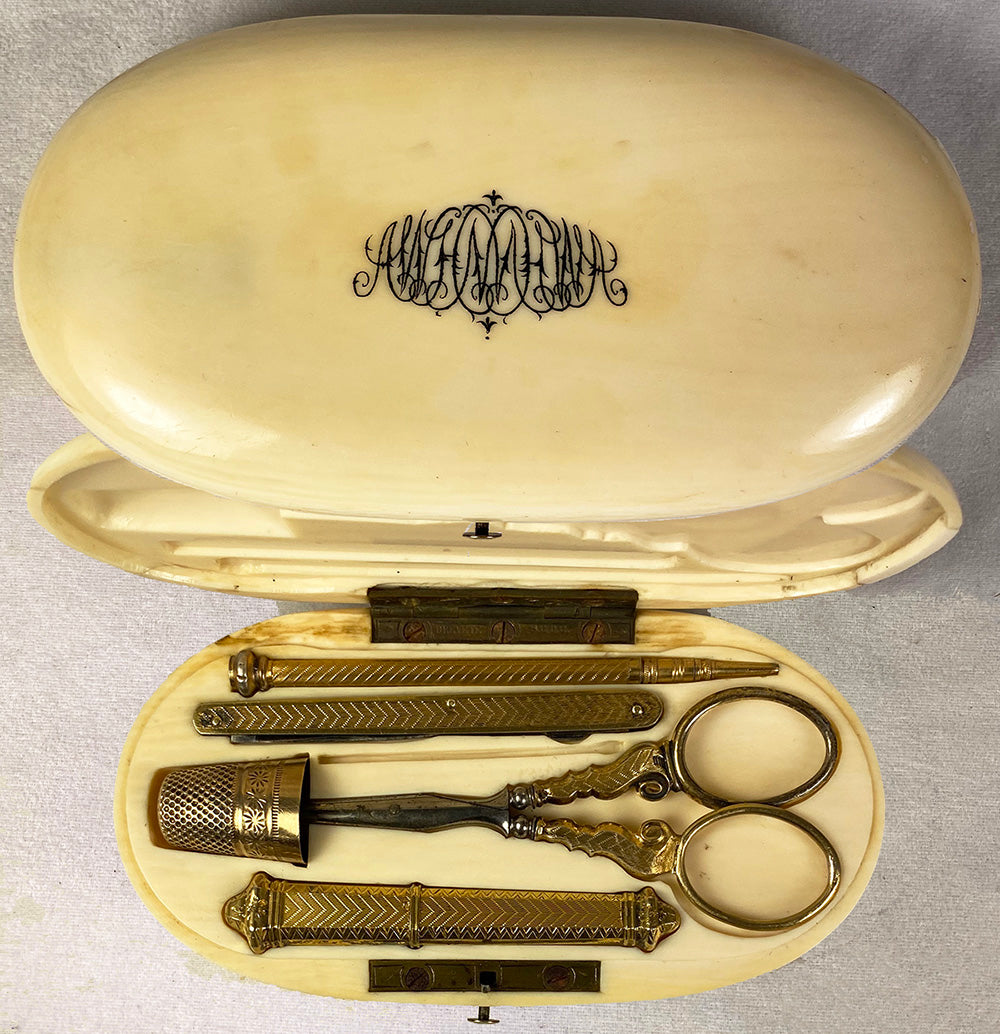This photograph depicts a vintage sewing kit housed in an ornate, oval-shaped hard case that resembles carved ivory or bone with a surface that mimics wood grain in an ivory cream color. The case features a decorative font and is shown both closed and open in the image. When open, the case reveals a carefully arranged set of faded golden brass tools, including a pair of small, fine-cutters scissors, a golden thimble reminiscent of the kind used in Monopoly, and potentially one or two sets of tweezers. Additional tools include what appears to be a long needle or file. These tools are neatly placed into specific indentations inside the exquisite, aged holder. The background of the image is white, ensuring all focus remains on the elegant sewing kit and its well-preserved contents.